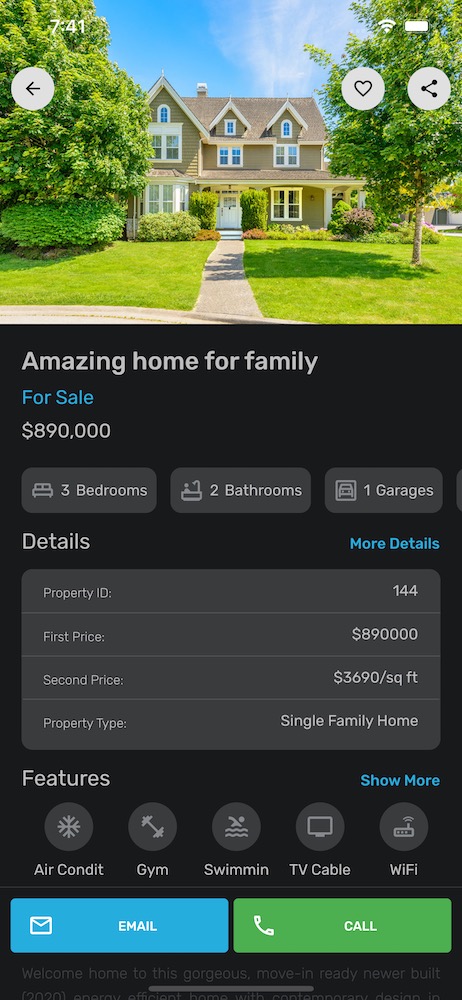**Detailed Caption:**

This screenshot was taken from an iPhone and displays the portrait mode view of a real estate listing. At the top of the screen, you can see the current time located in the upper left corner, along with the Wi-Fi symbol and a battery icon indicating the battery is almost fully charged. 

The main image is a three-story home, with the top-most story resembling an attic. The house is accessible via a paved sidewalk leading to the front door. The front yard is meticulously landscaped with well-maintained grass, various shrubs, and several trees on both the left and right sides of the house.

Below the image, there's a title that reads, "Amazing Home for Family." This home is listed for sale at a price of $890,000. Additional details are clearly outlined:
- Bedrooms: 3
- Bathrooms: 2
- Garage: 1
- Property ID: 144,000
- Price: $890,000 (First price), $3,690 per square foot (Second price)
- Property Type: Single Family Home

Further down, the features of the property are listed, which include air conditioning, a gym, a swimming pool, TV cable, and Wi-Fi.

At the bottom of the screenshot, there are two interactive buttons. The first button, labeled "Email," has a medium blue background with white text. An envelope icon is positioned to the left of the word "Email." To its right is a green button labeled "Call" in white text, featuring a white phone icon next to the word.